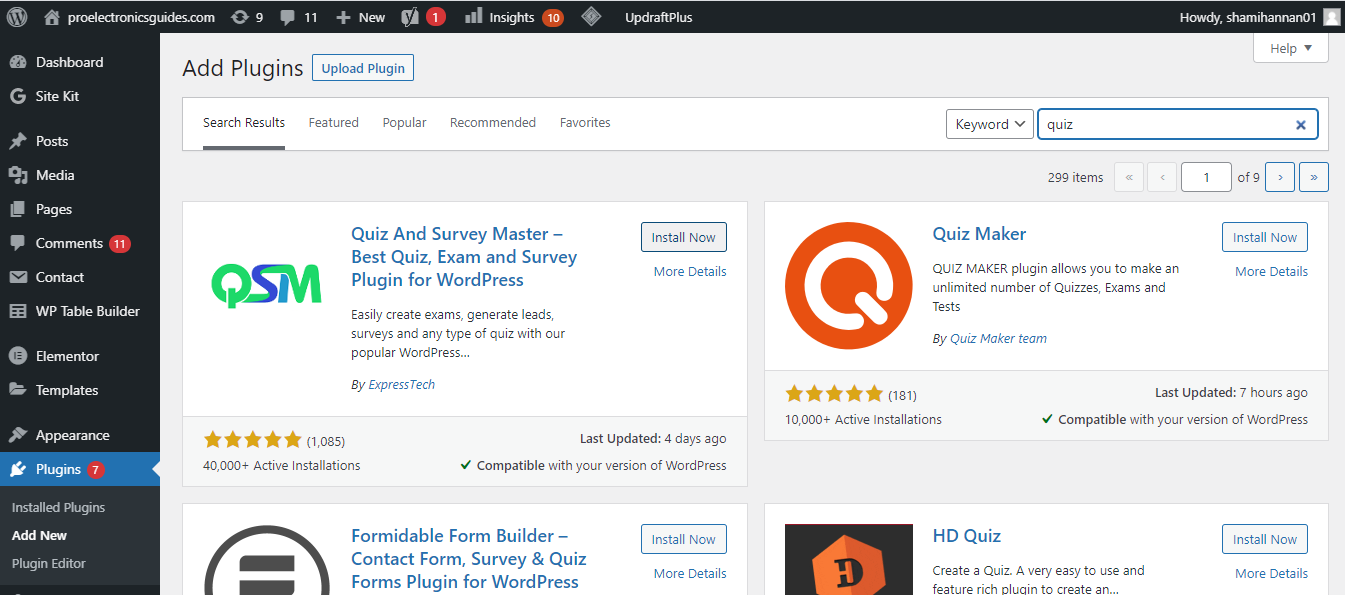This image is a screenshot featuring a user's WordPress admin dashboard interface, prominently set against a black background along the left and top edges. 

At the top of the screenshot, a round white circle with a 'W' logo is visible, followed by the text "ProElectronicsGuide.com" to the right. Below this header, the dashboard is divided into sections. 

On the left sidebar, key menu items are listed in white text including "Dashboard," "Site Kit," "Posts," "Media," "Pages," and "Comments" which has a red notification box showing '11'. Additional options like "Contact," "WPBuilder," "Elementor," "Templates," and "Appearance" are also displayed. The "Plugins" section is highlighted in blue, featuring a red notification box with the number '7'. Dropdown options under Plugins include "Installed Plugins," "Add New," and "Plugin Editor."

To the right of the sidebar, there is a white information box focused on the plugin "QSM" (Quiz and Survey Master). Written in green text is "QSM," followed by blue text indicating "Quiz and Survey Master, Best Quiz, Exam, and Survey Plugin for WordPress." An install button labeled "Install Now," located in the upper right corner of this box, is also noted. Directly below this description, a brief feature note reads "Easily Creates Exams."